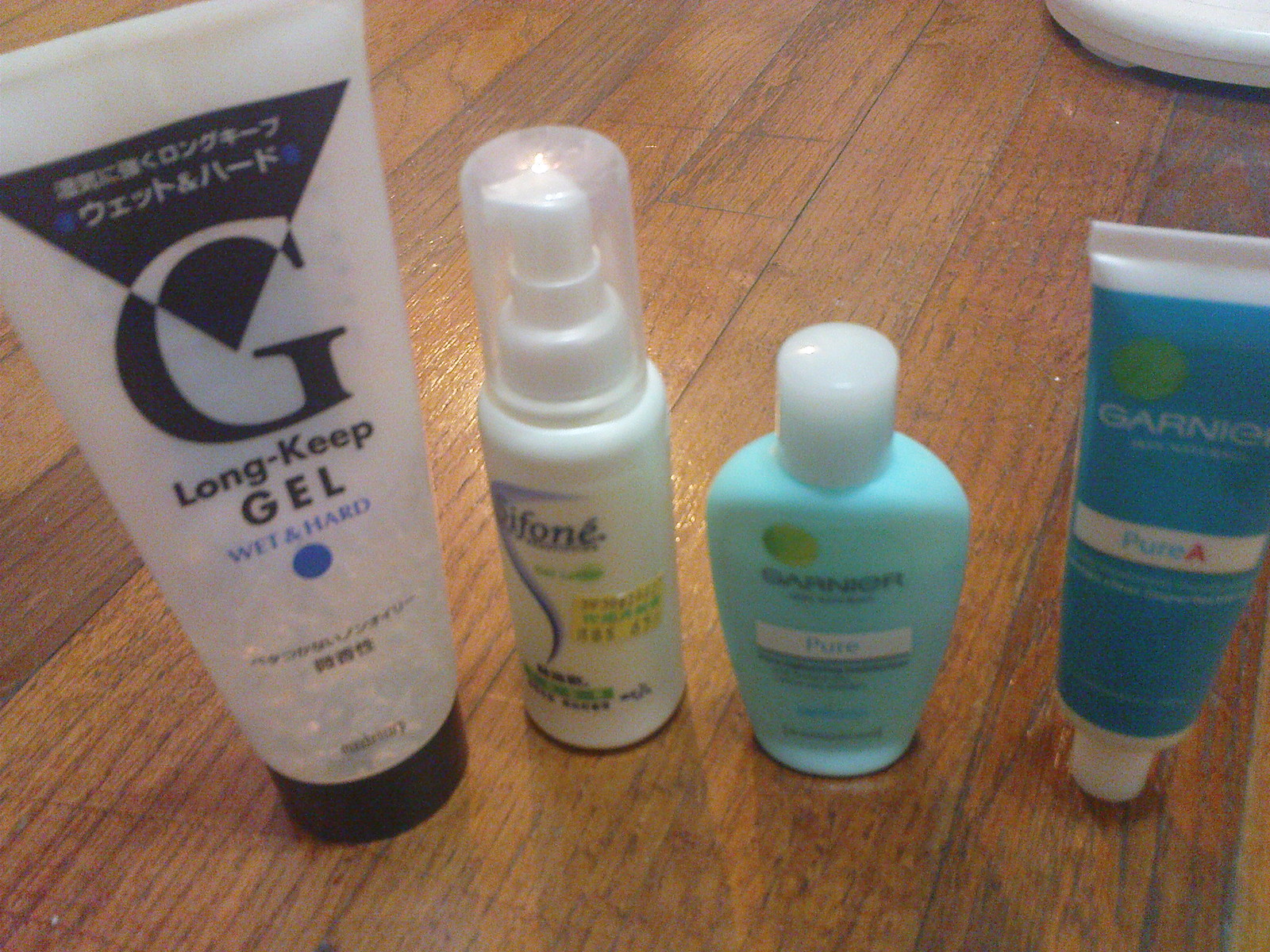The top-angle image showcases four personal care products laid out on a wooden surface, possibly a hardwood floor or a wooden table. At the leftmost position, there is a tall, clear bottle with a black cap, featuring the trademark G of Garnier. Below the G, the label reads "Long Keep Gel, Wet and Hard," adorned with additional non-English text. Adjacent to it is a smaller white bottle with a pump, marked by a yellow price tag and some foreign text; the label is partially readable and appears to say "Siphone" or "Biphone." Following this is a small teal bottle labeled "Garnier Pure." The final item on the right is another blue bottle, also from Garnier, marked "Pure A." The products are neatly positioned in the center of the image, set against shades of brown, white, black, blue, light blue, green, yellow, and red, indicating diverse packaging and possibly indoors with indeterminate lighting conditions.